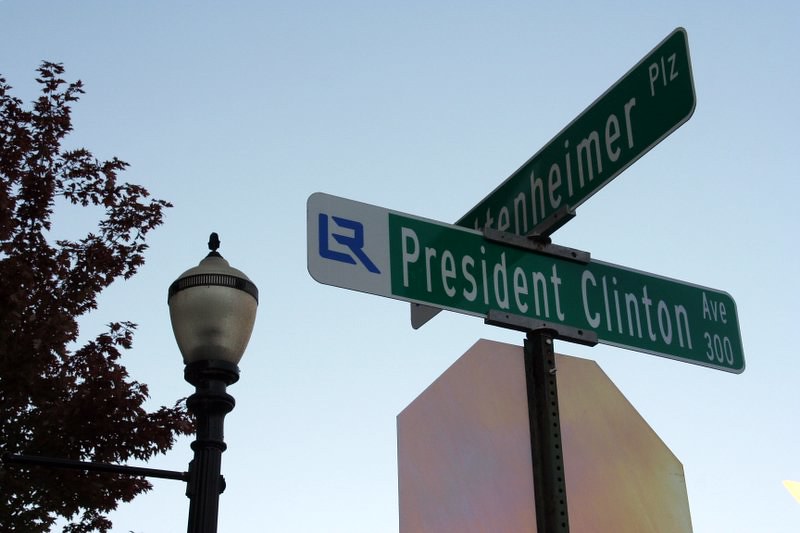This photograph, taken outdoors during what appears to be either late in the day or under dim lighting, captures a street sign on a pole slightly right of center against a pale blue sky. The image is horizontally oriented, making it wider than it is tall. Dominating the composition is a dual street sign on a metal pole, with the back of a stop sign partially visible on the opposite side of the pole.

In the foreground, the lower sign reads "President Clinton Avenue" with the number "300" situated in the bottom right corner, followed by a blue logo resembling "LR" on the left. Above it, another street name sign is partially visible; it reads "-ENHEIMER" and is accompanied by "PLZ" in the upper right corner, suggesting it could be something like "Eisenheimer Plaza."

To the left of the pole, there's a streetlight, and further left, a leafy tree extends into the frame, adding a touch of greenery. The subdued lighting and sky color hint that the photo might have been taken during the late afternoon or early evening, contributing to its serene urban atmosphere.